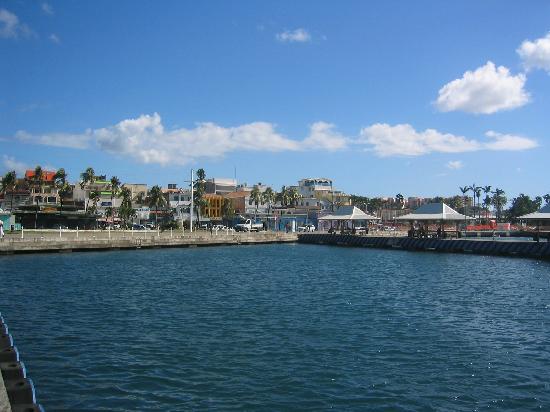The image captures a serene harbor scene, characterized by a vast, dark aqua-colored body of water occupying the lower 40% of the frame, with mild, consistent ripples. In the background, on the right-hand side, a dock stretches out while the left-hand side showcases a cement wall and walkway, flanked by two to three-story buildings. This appears to be a small town setting. Nestled behind the cement wall are commercial and residential buildings, some parked vehicles, and a few picnic tables under the pier areas. Further beyond, palm trees hint at a tropical locale. The sky above is a medium blue, adorned with a few picturesque, fluffy white clouds, completing the idyllic, sunlit harbor scene. No boats are present, but the infrastructure suggests a place designed for them to dock.